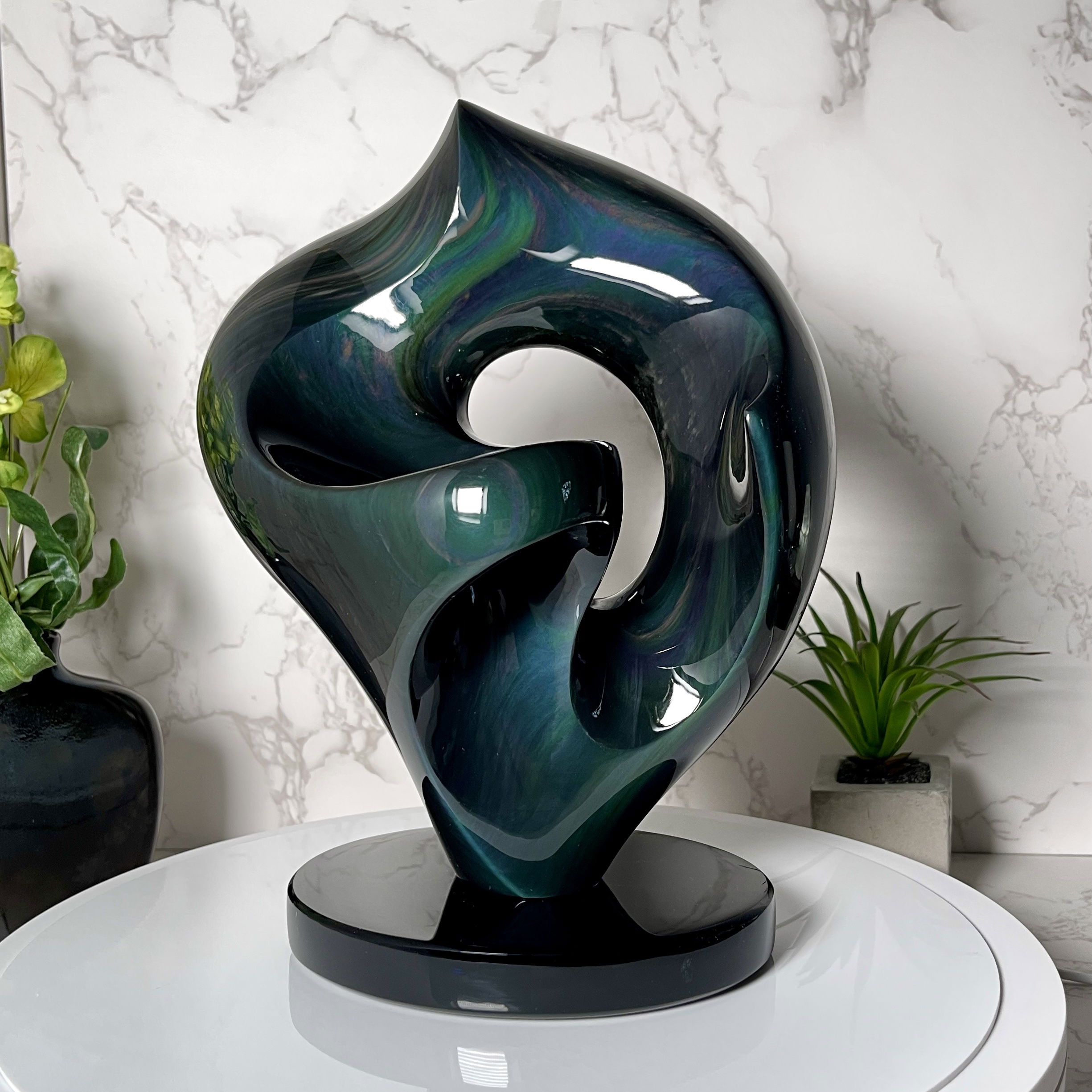The image depicts an elegant, abstract statuette with a distinctive and curvy form that resembles a heart or peach, yet is characterized by its smooth, asymmetrical shape which culminates in a point atop a circular black base. The statuette's surface features an eye-catching mix of oil slick colors, primarily deep blues and greens with occasional hints of purple, giving it a marble-like texture. It stands prominently on a pristine, white round table set against a sophisticated backdrop of a white marble wall with grey marbling.

To the right of the statuette is a small succulent plant housed in a cement square container, while to the left, there is another large, dark-colored vase, possibly black or a deep greenish-blue, containing additional plant fronds. The entire setting exudes a sense of refined elegance and artistic flair, making the statuette the focal point of this aesthetically pleasing arrangement.